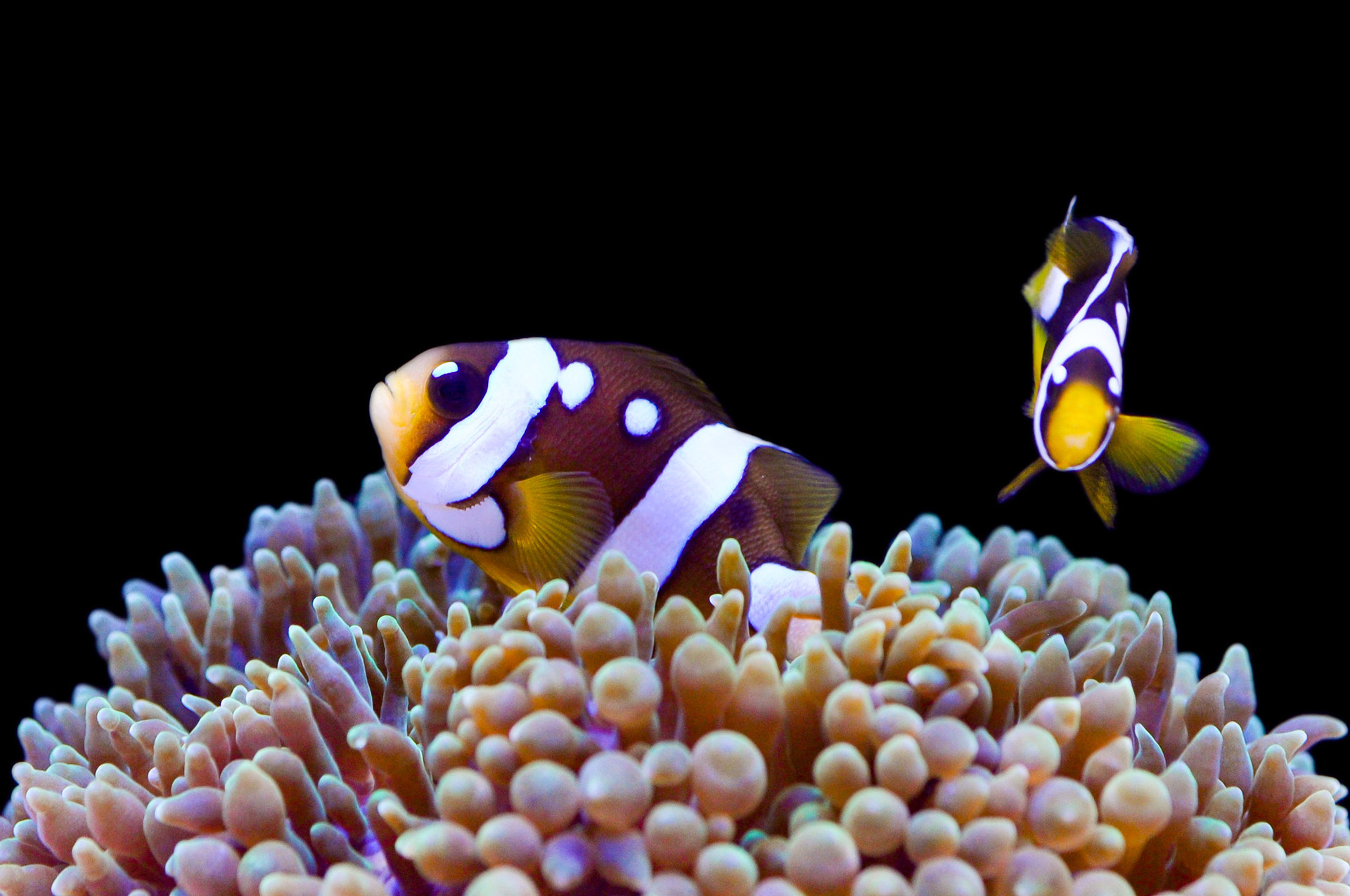The photograph captures a pair of nearly identical tropical fish swimming in an underwater setting against a pitch-black background. Both fish are characterized by their mostly brown bodies, adorned with two prominent white stripes and two white dots near the top. Their large black eyes contrast with their white mouths. The fish also feature vibrant yellow fins that are tipped with blue, adding a colorful detail to their appearance.

The fish on the left is partially concealed by a sea plant, which is shaped like a half circle and has various worm-like, brownish tendrils. It looks leftwards while peeking out from the plant. Meanwhile, the right fish faces directly forward, making their different orientations quite noticeable. The close-up nature of the photograph accentuates the fish's bright colors and intricate details, highlighting their vibrant and tropical aesthetic, even more, against the stark, black background.